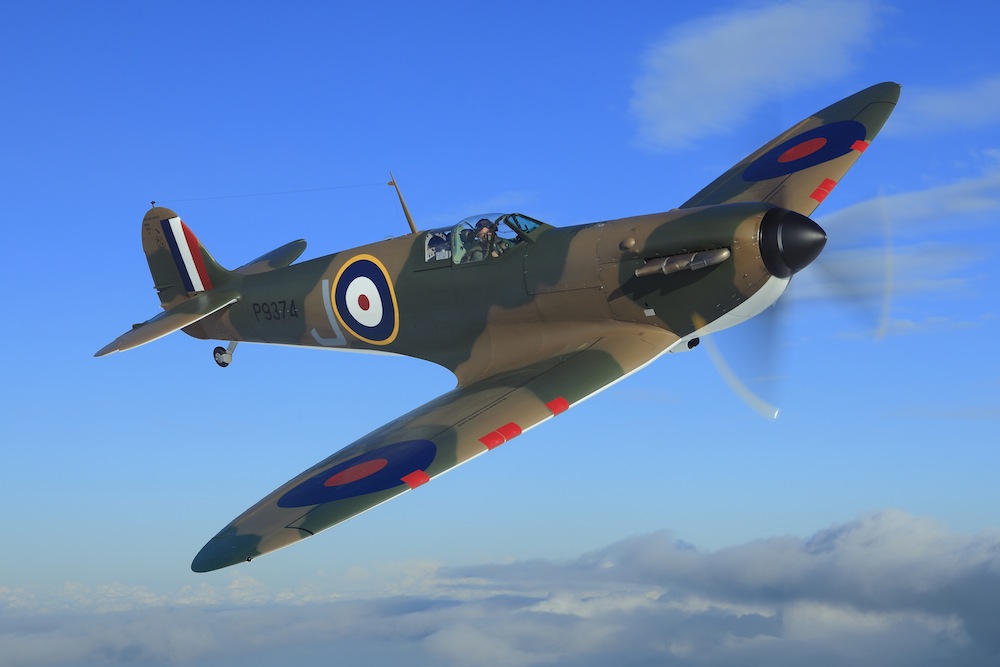This is a 3D-rendered image of a classic Supermarine Spitfire flying high above the clouds on a bright blue day. The single-engine, camouflage green and tan plane is diagonally oriented with the left wing higher than the right. Its black nose cone and rapidly spinning propeller blur into the background. The fuselage features a prominent bullseye emblem with concentric rings—yellow on the outermost, followed by dark blue, white, and a red center. Each wing also displays a similar bullseye, with blue outer circles and red centers, interspersed with small red squares forming a pattern. The tail of the plane carries a blue, white, and red striped marking. A single male pilot is visible in the clear bubble cockpit, donned in a green army uniform and helmet. The side of the aircraft is marked with "P9374" and a large "J" positioned next to the bullseye symbol. The sky backdrop is adorned with wispy, light gray clouds at the top and a thicker layer of darker clouds extending from the bottom left to the bottom right, contributing to the overall serene yet dynamic aerial scene.